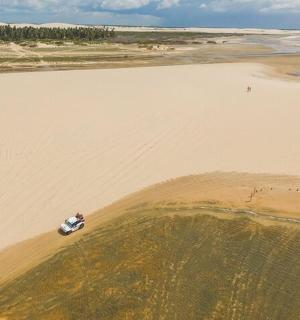This is a small, square, aerial photograph capturing a beach scene. The central focus is a body of water, which appears extremely dirty and is a light tan color due to the high presence of dirt. This stretch of murky water horizontally divides the image. Bordering the water is a narrow strip of darker tan sand, forming the beach. 

Parked close to the water's edge on the beach is a white vehicle, likely a sedan or hatchback, with a brown object sticking out of its back. Adjacent to the beach, on one side of the water, lies a green lawn with patches of dead brown grass. On the opposite side, the scene transitions into another sandy area, which features a line of spiny-leafed trees below a partly cloudy, blue sky. Towards the top left of the image, there are scattered trees, while the far right shows the edge of the water starting to advance as the tide comes in.